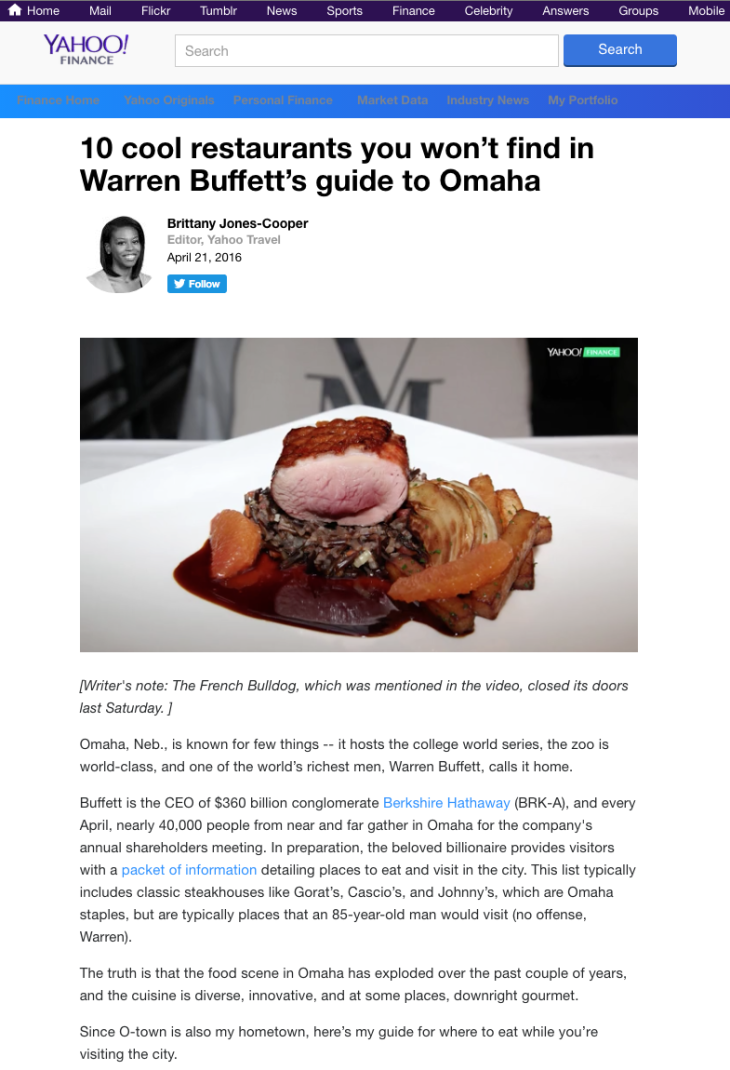### Detailed Caption for Screenshot from Yahoo Finance Website

This screenshot is taken from the Yahoo Finance section, showcasing a comprehensive and neatly organized layout. At the top, a dark blue navigation bar features various options including Home, Mail, Flickr, Tumblr, News, Sports, Finance, Celebrity, Answers, Groups, and Mobile, providing quick access to different segments of Yahoo. Below this bar, the Yahoo Finance logo is prominently displayed next to a search bar, enabling users to easily search for financial information.

A bright blue secondary navigation bar is positioned under the search bar, offering specific categories such as Finance Home, Yahoo Originals, Personal Finance, Market Data, Industry News, and My Portfolio. This helps users navigate through different sections of the finance website efficiently.

The centerpiece of the page is an article titled "10 Cool Restaurants You Won't Find in Warren Buffett's Guide to Omaha," presented in bold black text. The article is authored by Brittany Jones-Cooper, identified as an Editor for Yahoo Travel. A black and white photo of the young, smiling author is included next to her name, along with her job title. The publication date, April 21, 2016, is clearly mentioned, and a blue Twitter follow icon is provided for readers to connect with the author on social media.

Below the article title, a captivating image of an upscale restaurant meal hints at the ensuing content. A notable writer's note follows, indicating that The French Bulldog, one of the mentioned restaurants, had closed its doors the previous Saturday.

The article itself begins by highlighting Omaha, Nebraska's well-known features such as hosting the College World Series, its world-class zoo, and being home to one of the world's richest men, Warren Buffett. It outlines Buffett's role as CEO of Berkshire Hathaway and the annual pilgrimage of nearly 40,000 people to Omaha for the company's shareholders meeting. Buffett provides visitors with a curated list of places to eat, generally including classic steakhouses that are favorites of an 85-year-old man, like Gort's, Casio's, and Johnny's.

However, the article's purpose is to reveal that Omaha's food scene has evolved dramatically, offering a range of diverse, innovative, and gourmet cuisine. The author, who is also a native of Omaha, shares her personal recommendations for dining in the city, providing an alternative guide for visitors.

This detailed caption encapsulates the structure and content of the Yahoo Finance webpage, providing a vivid and complete description.